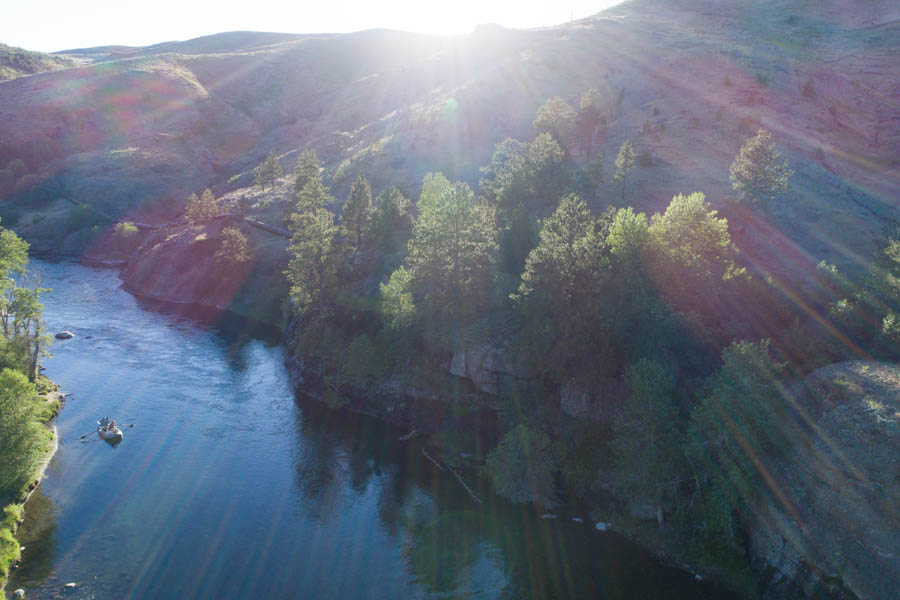A breathtaking landscape photograph captured in the early morning as the sun rises over distant mountains. The powerful sun rays bathe the entire scene, casting a bright light that fades the colors into soft tones of red, dark green, and light green. The scene features a winding river that flows from the center left towards the bottom right of the image, its waters appearing slightly dark and interspersed with sticks and rocks. Nestled on the river is a small boat or canoe, positioned near the left side. On the bank, to the left center of the image, are delicate, wispy green leaves of trees, while darker boulders and rock formations dominate the bottom right. Pine or evergreen trees border the river, growing amidst the rocky shores. This harmonious blend of natural elements, accentuated by the dramatic sunlight, creates an awe-inspiring outdoor vista.